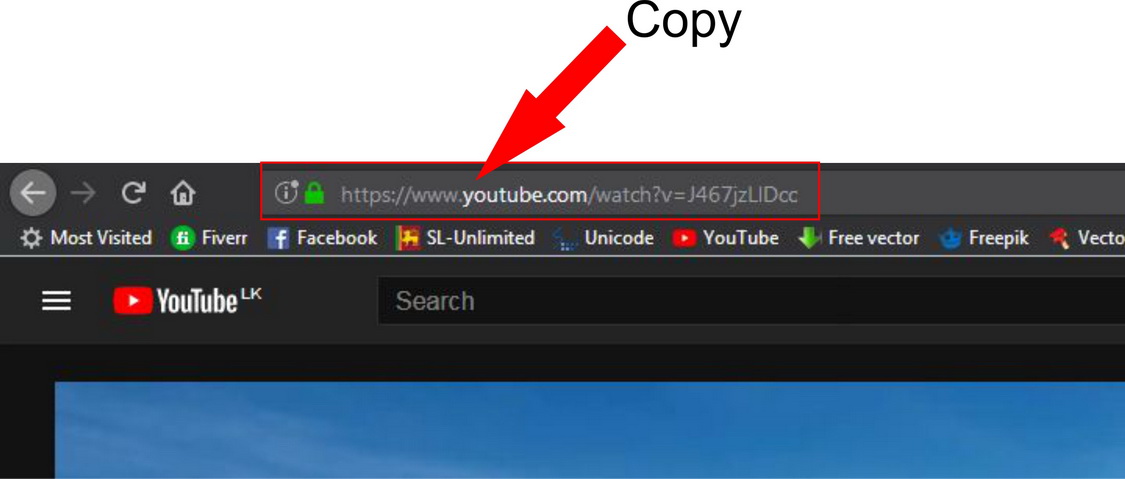The image is a screenshot of a web browser in dark mode, featuring a predominantly dark gray and black color scheme. At the top left of the browser, there is a white left-arrow icon encircled in gray, followed by a plain gray right-arrow icon. Next to these navigation controls, there is a white refresh icon shaped like a semicircle, and beside it, an icon resembling a small house, symbolizing the home button. 

The address bar is gray and contains a few icons: a gray circle with an eye inside, a green lock icon, and the URL "https://www.youtube.com/watch?v=J467JZLIDCC" in gray text. 

Above the address bar, the top portion of the screenshot is white with a large red arrow pointing towards the YouTube logo. The arrow is labeled with black text reading "copy."

Below the address bar, there is a toolbar displaying recently visited websites and bookmarks, including "Most Visited," "Fiverr," "Facebook," "STL Unlimited," "Unicode," "YouTube," "Free Vector," "Free Pick," and partially visible "VectO."

In the main content area, the first element from the left is a menu icon represented by three horizontal lines. Next to it is the YouTube icon, which is a red play button with a white triangle in the center. Adjacent to this is the text "YouTube" followed by "UK" in lowercase letters. 

Underneath, there is a large search bar with a black background and gray text that reads "Search." Below the search bar is another black border, which frames a blue screen occupying the remaining section of the screenshot.